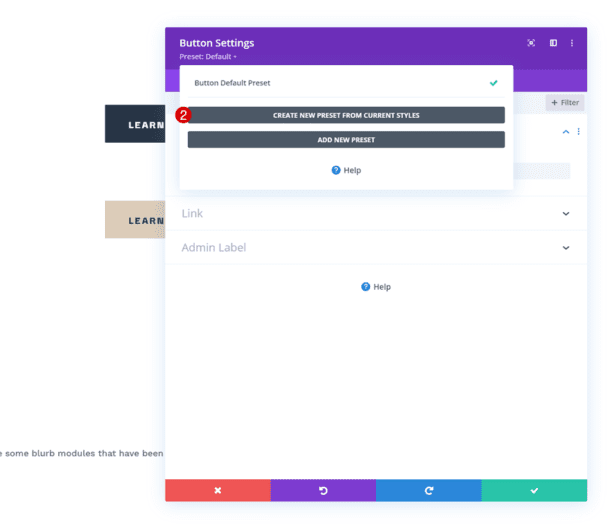The image depicts a cascading series of dialogues layered atop one another, with each layer progressively more prominent and complex. 

In the background, there is a relatively small dialogue box featuring three distinct panels: a grey one, a white one, and a cream-colored one. These panels form a foundational layer, subtly adding depth to the composition.

Directly above this foundational layer is a significantly larger dialogue box adorned with a prominent purple banner across the top. This banner references button settings and the preset default, setting a technical and functional tone. Towards the right side of this dialogue, there is text indicating a filter function. The box also includes a link pull-down menu and an admin label pull-down menu. Centrally located is a blue help button, easily accessible for assistance. At the bottom of this dialogue box are four mini-panels, each with distinct colors and icons: a red "X" for closing, a purple circular arrow for resetting, a blue circular arrow pointing in the reverse direction for undoing actions, and a green tick mark signifying confirmation or approval.

At the forefront of this layered arrangement is a third, predominantly white dialogue box, overlaying the other two. This box features two elongated grey buttons. The first button, marked with a red numeral "2" on the left, is labeled "Create new preset from current styles." The second button is labeled "Add new presets." At the top, this dialogue mentions "Button Default Preset." Like the previous dialogue, it also includes a central help option for user guidance.

The image intricately combines these dialogues, creating a visually complex yet organized structure, each layer fulfilling a specific role in the user interface.